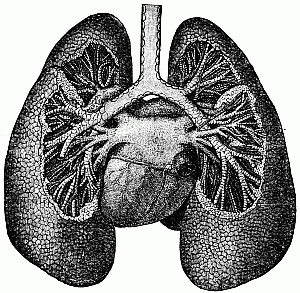This is a detailed black and white diagram of the human respiratory and circulatory systems, focusing primarily on the lungs and heart. Drawn in a rectangular shape with a plain white background, the image showcases both lungs and their intricate internal structures. The windpipe or trachea is seen leading into the lungs, which are depicted in a cross-sectional view to reveal the branching airway passages. Central to the illustration, the heart is situated between the lungs, with arteries and veins visibly connecting between the heart and lungs, highlighting the circulatory pathways. The entire drawing, rendered in black ink or pencil, provides a clear and meticulous look at these vital organs and their interconnections.